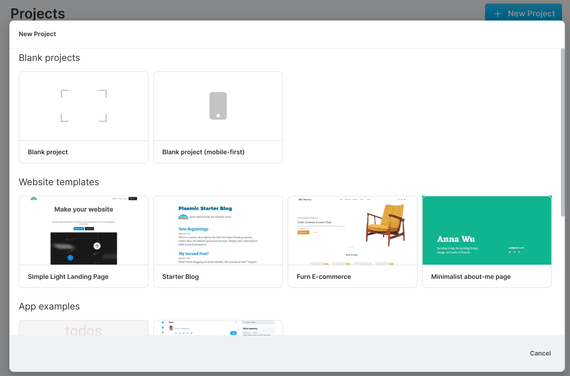This image is a screenshot of a computer interface, likely a project management or design platform. The layout features a clean white background with a subtle gray border. 

In the upper left corner, there is a black header titled "Projects." Below this, the main content area lists various project options. The first section includes two outlined squares: 
1. The first square has a text label "New Project" and is marked by a dashed border, implying it's a clickable area to initiate a new project.
2. To the right of this, there is another white square featuring a phone icon with the label "Blank Project, Mobile First," suggesting this option is for mobile-oriented projects.

Further down, the section titled "Website Templates" presents four horizontal rectangular options:
1. The first rectangle, labeled "Make Your Website," displays an icon of a computer screen.
2. The second rectangle is labeled "Starter Blog," intended for creating a blog.
3. The third rectangle shows an image of a wooden chair with a yellow cushion and some accompanying text on its left side.
4. The fourth and final rectangle is green with the name "Anna Wu" inscribed on it, though its specific purpose is unclear.

Overall, this interface appears to be designed for users to select and initiate different types of projects, from new designs to specific templates.